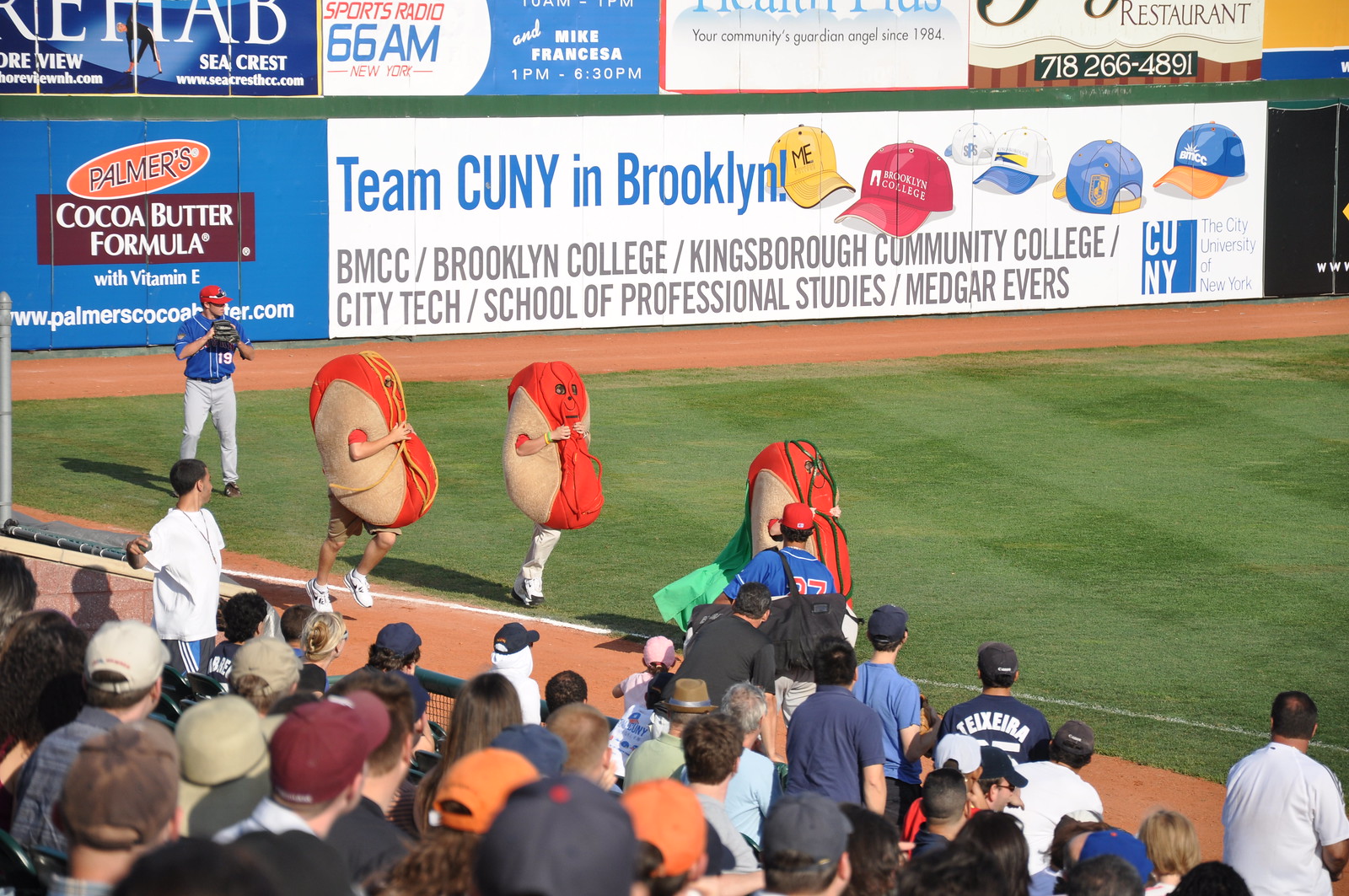This detailed horizontal photograph captures an energetic moment at what appears to be a professional baseball game in the late afternoon. The image is taken from the stands, showcasing the backs of numerous spectators who are all standing and intently watching the scene unfold on the vibrant green field. Prominently featured along the sideline, and evoking a playful atmosphere, are three individuals dressed in whimsical hot dog costumes; each costume consists of a red wiener encased by buns, with the wearers' arms and legs visible. Among them, also near the sideline, stands a photographer, busy capturing the event.

Beyond the costumed characters, a baseball player dressed in a blue jersey, gray pants, and a red hat is visible. He is poised with a pitcher's glove, ready to throw. The field's edge is marked by a strip of dirt, indicative of a baseball diamond. In the backdrop, a sizable advertisement wall is filled with various sponsor logos, including a prominent ad for Palmer's Cocoa Butter Formula and another for Team CUNY in Brooklyn, listing different colleges like BMCC, Kingsborough Community College, City Tech, School of Professional Studies, and Medgar Evers College. These details collectively suggest a lively and engaging baseball event, possibly linked with the City University of New York.